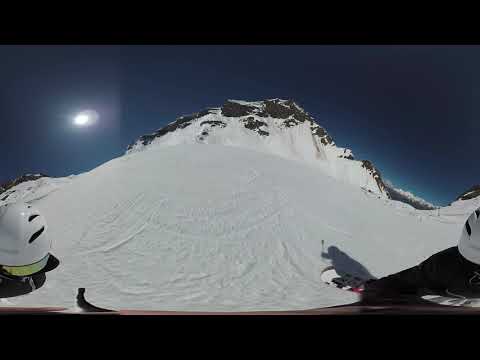This vibrant 360-degree daytime image captures a dramatic snow-covered mountain scene with a clear, deep blue sky. The sun peeks through the upper left-hand corner, casting a warm glow over the snowy landscape. The mountain, prominently featured in the middle top of the image with its gray, bare peak, contrasts beautifully with the dense blanket of snow covering its slopes.

In the foreground, two helmets are visible at the edges of the image—a white ski or snowboard helmet with black vents, a yellow visor, and black straps positioned on the bottom left, and another matching helmet on the bottom right. A shadowy figure, holding what appears to be a ski pole or snowboard stick, is faintly visible to the right, casting a dark silhouette on the snowy ground. Additionally, a ski or snowboard with white and red coloring is seen at the bottom right, paired with black pants, reinforcing the winter sport activity. The image showcases an adventurous moment, likely of skiing or snowboarding, against the stunning backdrop of majestic, snow-laden mountains.